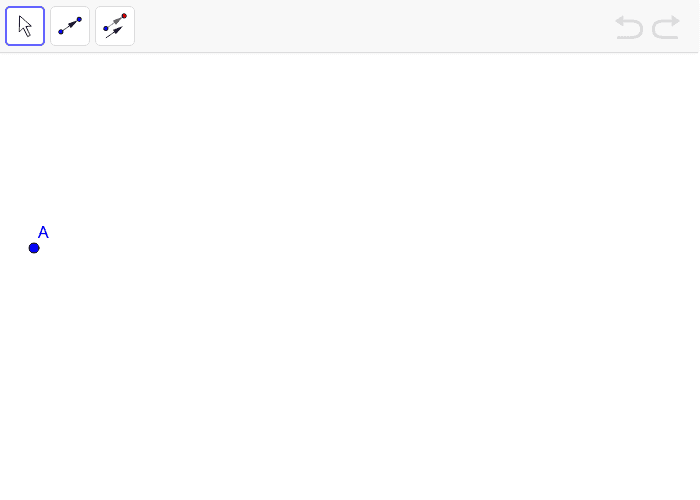At the top of the image, there is a long gray bar. On the far left side of this bar, a square is outlined in blue, containing an upward and leftward-pointing white arrow, outlined in black and diagonally centered. To the right of this blue-outlined square, there is another square outlined in light gray, featuring two small dots and an arrow pointing toward the right dot. Next, there is a third square also outlined in light gray; it displays a blue circle on one side and a red circle on the other side. This section of the bar is relatively short, around two to three inches long, with an arrow pointing to the right positioned underneath. This arrow measures about two inches in length. Approximately five inches further to the right within this gray rectangle, there is another arrow that curves upward and points to the left, alongside an arrow starting from the bottom that curves up and to the right. Both of these arrows are depicted in a light gray color.

Moving down to the left side of the image, about four inches below the top bar, there is an uppercase letter "A" in blue, standing about one inch tall. Beneath this letter "A" is a blue dot approximately half an inch in height.